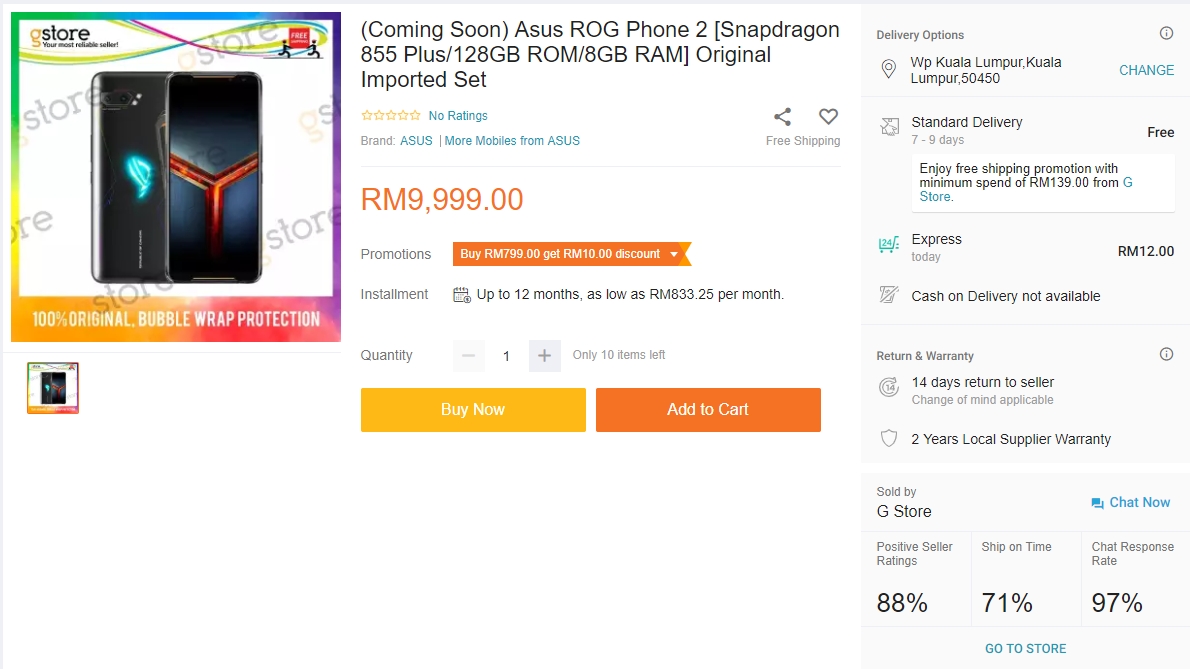The image showcases a screenshot of a shopping app, prominently featuring a product listing for the ASUS ROG Phone 2. On the left side of the screen, there is an image of the phone. Beneath this image, a caption reads, "100% original bubble protection." The product description notes that it is "coming soon" and details the phone's specifications as "ASUS ROG Phone 2 [Snapdragon 855 Plus / 128 GB ROM / 8 GB RAM] original imported set." The listed price for this product is RM 9,999.00.